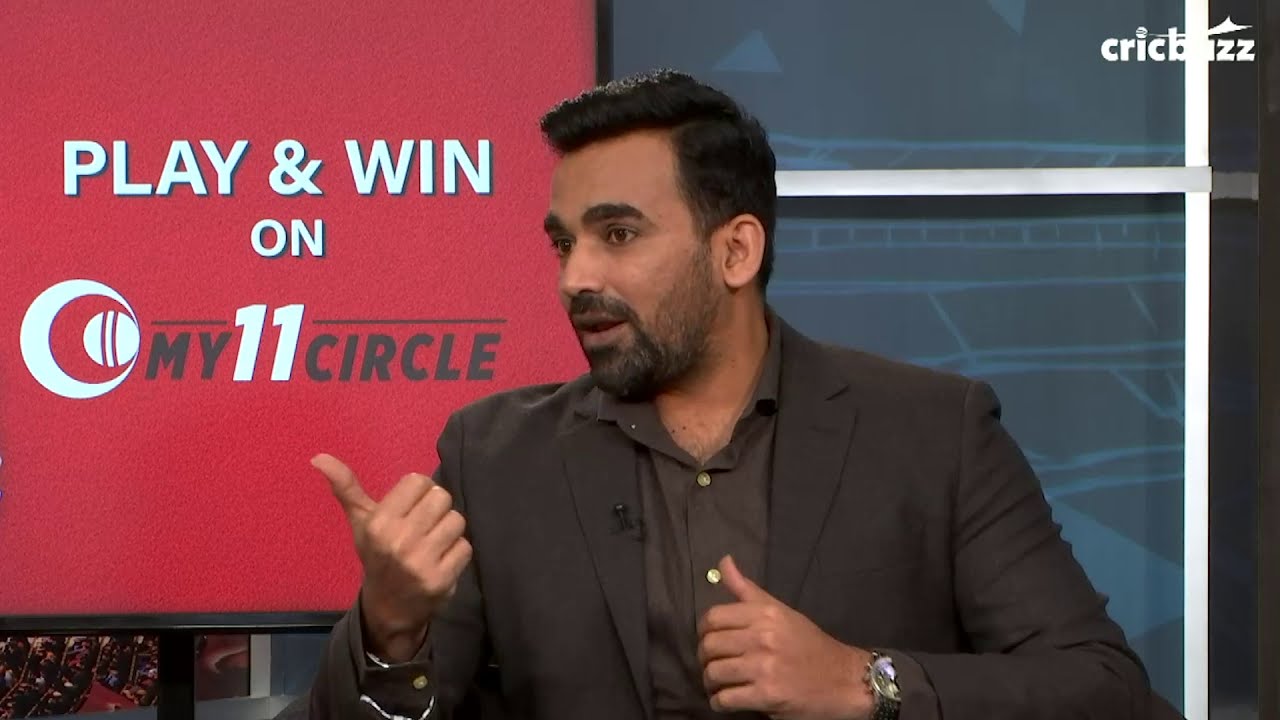The image is a screenshot from a sports television program. It features a man in his 30s with dark hair, slightly balding, combed and slicked back in a part. He has an olive complexion, a scruffy beard and mustache, and a five o'clock shadow. He is wearing a dark brown suit with a matching dark brown button-up shirt. A lapel mic is pinned to his right lapel, and he has a watch on his left wrist. The man is seen talking animatedly, gesturing with his right hand and looking off to the left side of the image.

In the background, a red sign prominently displays the text "play and win on my 11 circle," accompanied by a logo featuring a ball inside a crescent moon. In the upper right corner, there is text that reads "Crick Buzz" (C-R-I-C-B-U-Z-Z) with a small swoosh above it. The background also features an illustrated depiction of an arena, emphasizing the sports theme of the program.